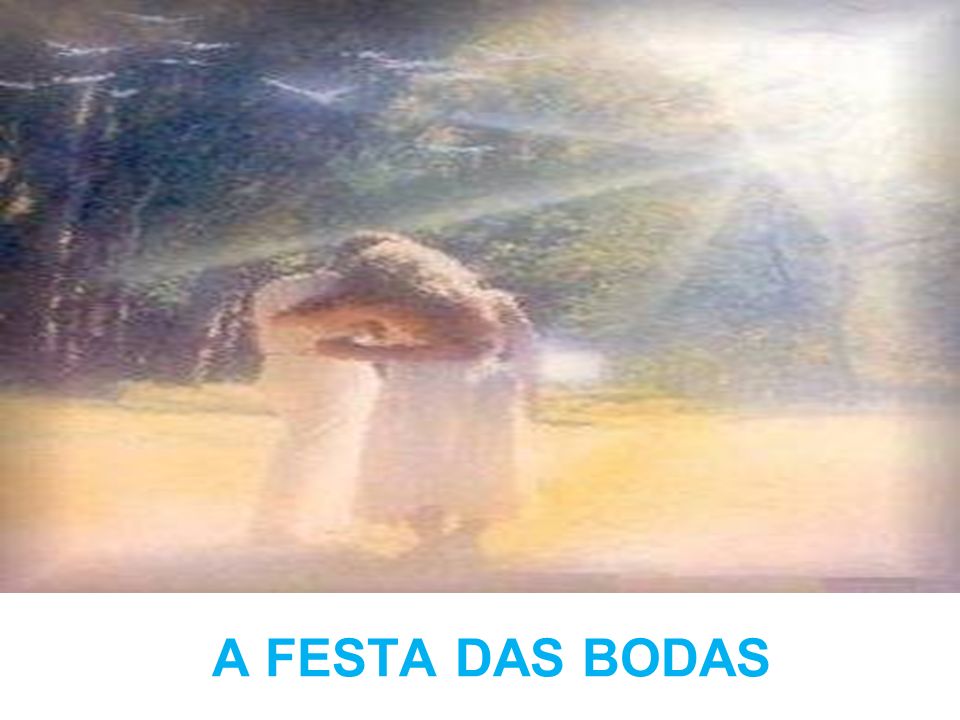In this blurred and weathered rectangular photograph, a man and a woman dressed in white embrace each other while standing in the center of a large sunny field. The background features an overexposed sun in the upper right-hand corner, casting a bright light that distorts the image, and trees on the left side. The ground beneath them is a yellowish-tan, resembling a sun-bleached field rather than green grass. The faded quality of the photograph gives it an old, nostalgic feel, reminiscent of 1980s magazine imagery. At the bottom of the image, the text "a festa das bodas" is written in blue font against a white background, suggesting a romantic or celebratory theme in a language that appears to be Portuguese.